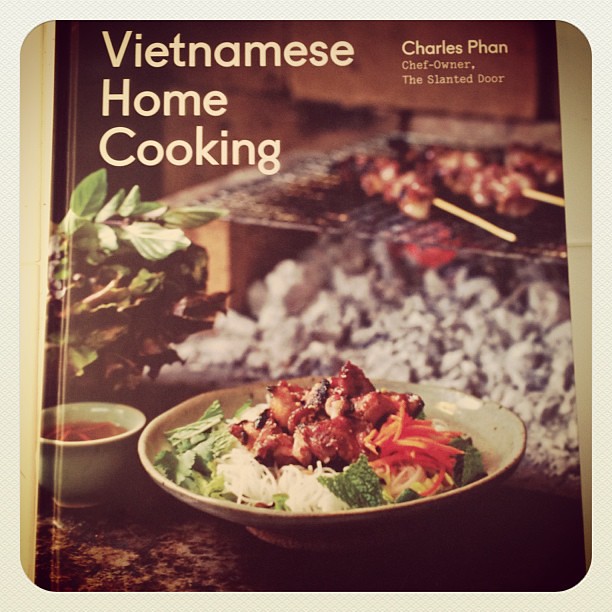A vibrant photograph depicts the front cover of a cookbook titled "Vietnamese Home Cooking" by chef-owner Charles Phan of The Slanted Door. The square-shaped cover features rounded edges and a rich array of colors including red, orange, yellow, white, green, brown, beige, tan, and black. In white letters, the title "Vietnamese Home Cooking" is prominently positioned in the top left corner, while Charles Phan's name appears to the right in smaller text.

Dominating the lower portion of the cover, a bowl brimming with a variety of ingredients catches the eye. It contains a medley of vegetables, noodles, and different meats, complemented by a small bowl of sauce to its left and some lettuce positioned behind it. Adding to the cover’s allure, the background showcases a slightly blurred image of meats skewered on sticks, being grilled over coals, reminiscent of a traditional hibachi setup. 

Overall, this detailed and colorful image emphasizes the culinary expertise and inviting flavors featured in Charles Phan's cookbook.